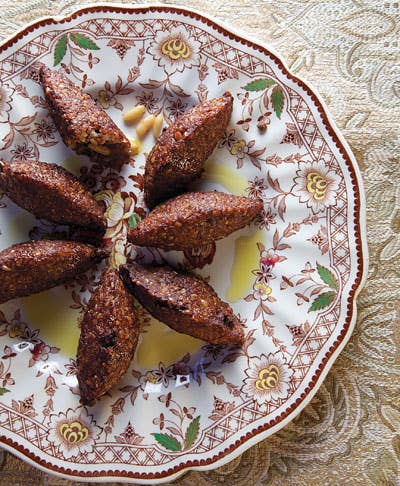The image showcases a beautifully arranged dish of food on a decorated china plate, which rests on an ornately patterned floral tablecloth. The plate itself features a maroon and green floral print with a checkered border, scalloped rim, and red lining, suggesting an expensive and ornamental design. The food, of an oblong shape and dark maroon or brown color, presents an intriguing display. Surrounding the central food item are a few specks of rice, numbering seven and arranged in a star-like pattern facing outward. A layer of yellow oil beneath the food hints at it being baked. Pine nuts are scattered atop the plate, adding a final touch to the visually appealing presentation. The overall image, captured in vibrant colors, emphasizes the effort and cultural significance behind the meal, making it suitable for a food blog, magazine, or someone's personal collection.